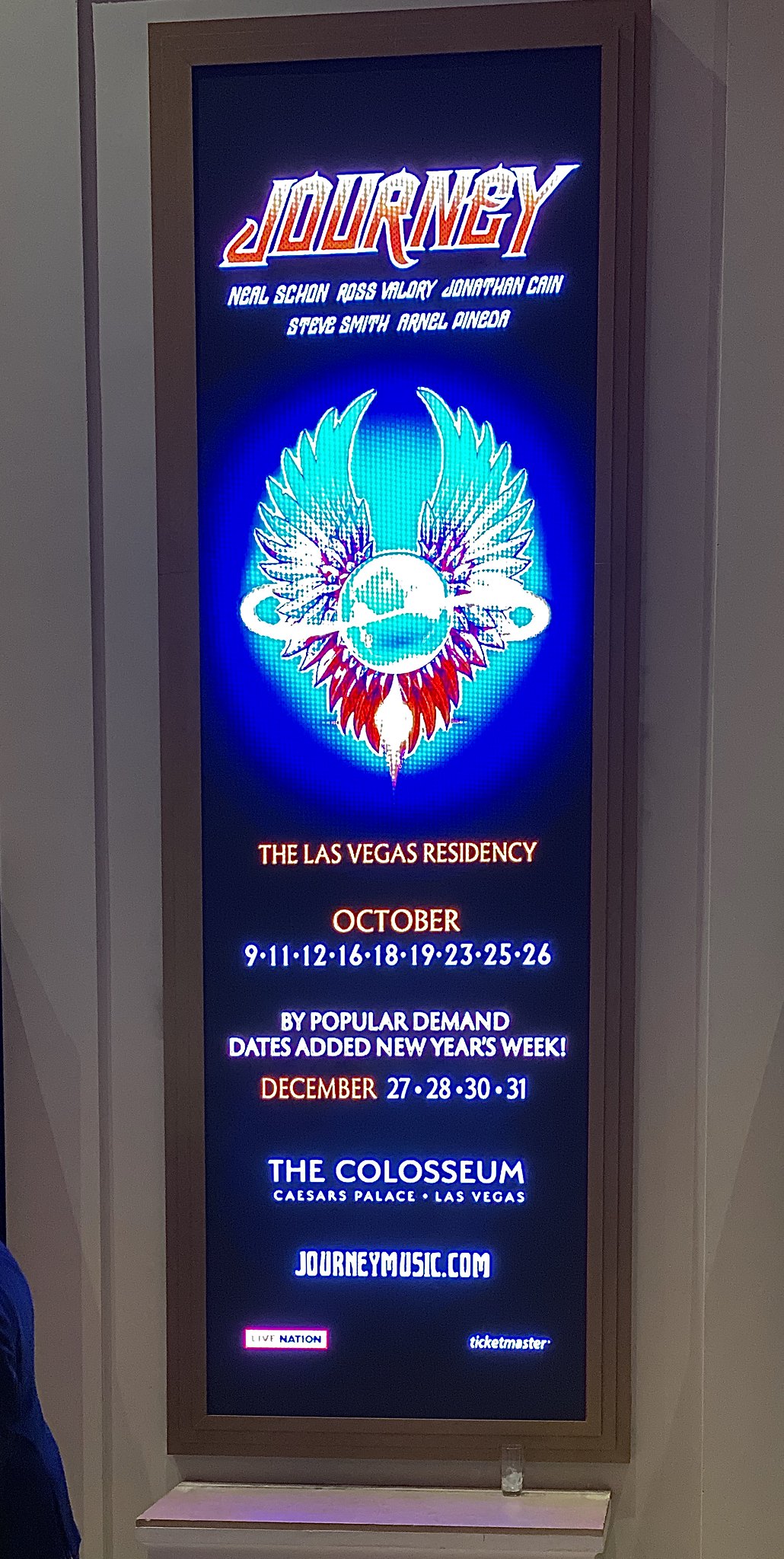The image is a detailed color photograph of a vertical LED banner, prominently displayed on a white wall and artistically framed with a dark brown wooden border. This backlit billboard, typical of a theater lobby or concert venue, showcases an advertisement with a black background and vibrant graphic design elements. At the top, the banner features the iconic logo of the band "Journey" in a gradient that transitions from yellow to red. Below the band's name, two lines of white text list the members: Neil Sean, Ross Valerie, Jonathan Cain, Steve Smith, and Arnel Pineda. Central to the design is the band's emblem — a sphere with sprawling wings that boast a patriotic color scheme: blue at the tips, white in the middle, and red at the base, all against a radial gradient backdrop that fades from dark blue to aqua. Further down in bold yellow text, the banner advertises "The Las Vegas Residency," followed by "October" and a list of dates: 9, 11, 12, 16, 18, 19, 23, 25, and 26. Additional white text at the bottom announces extra performances by popular demand for New Year's week, followed by location details at "The Coliseum Caesars Palace Las Vegas," and the band's website, "Journeymusic.com". This meticulous composition is a prime example of graphic design utilized in advertising.